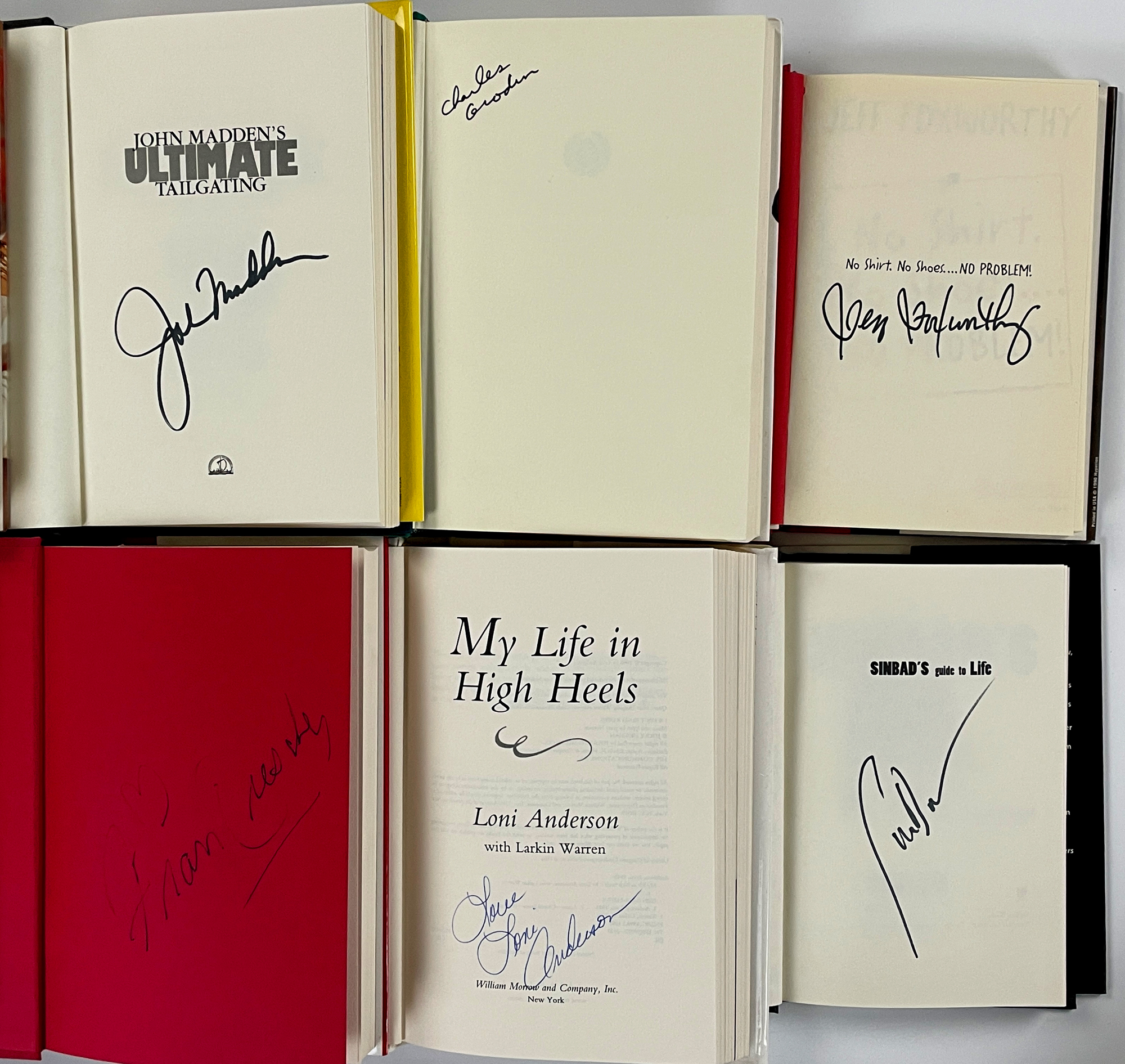This photograph captures a collection of six open books, each featuring a signed interior cover or title page. The books, which are arranged in a squared perspective, include notable titles and signatures from famous personalities, mainly actors, comedians, and TV personalities. In the upper left, there is "John Madden's Ultimate Tailgating" signed by John Madden himself. Another is "No Shirt, No Shoes, No Problem," although the author’s signature is unreadable. Following the sequence, an unnamed red-covered book also contains an indecipherable signature. "My Life in High Heels" by Lonnie Anderson, co-authored with Larkin Warren, prominently displays Lonnie Anderson's signature in blue ink along with a message. The last book visible in the assortment is "Sinbad's Guide to Life," which also features his signature. The primary colors observed in the image are red, white, black, and yellow.